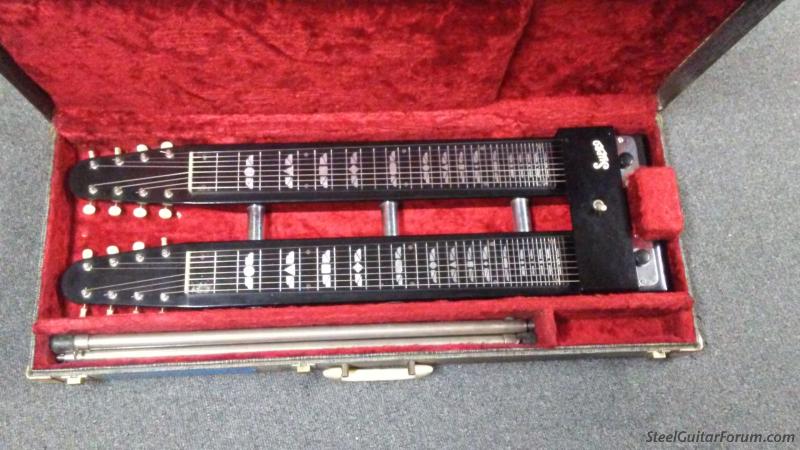The horizontally rectangular, full-color photograph, shot outdoors in natural daylight, depicts an opened rectangular case resting on a gray, textured sidewalk. The unbordered image prominently features a luxurious red velvet-lined interior, showcasing two wooden, eight-string musical instruments. These instruments, likely some variation of a steel guitar, are securely nestled within designated slots, complete with visible silver strings and black bases. The lids open to reveal the tuning pegs and bars upon which the strings rest. Positioned at the bottom of the case is a narrow compartment containing two metallic rods of unspecified use. Black text in the lower right corner reads "SteelGuitarForum.com," providing a clear attribution.